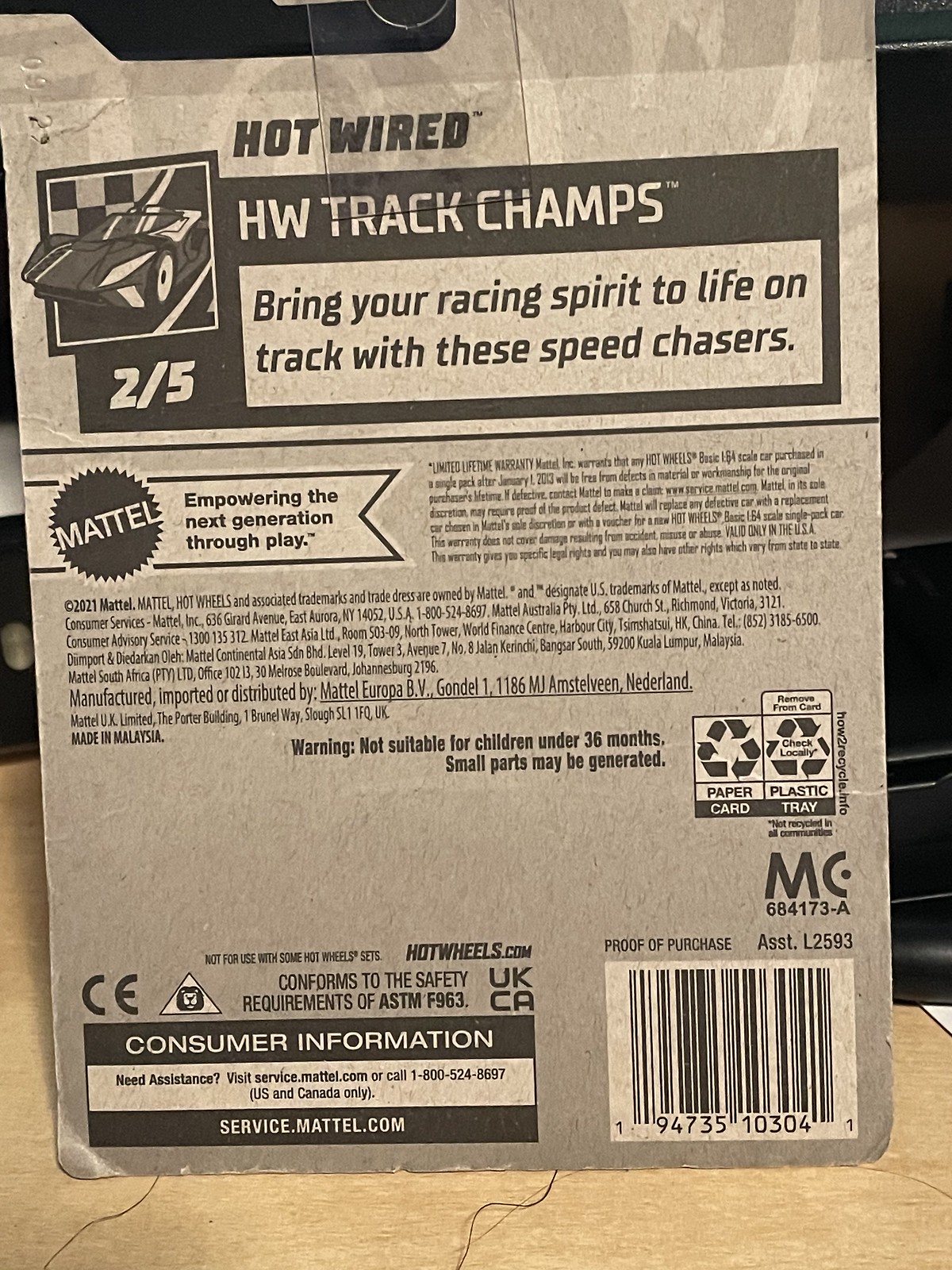This tall rectangular image depicts the back of a toy car package set against a light brown wooden surface. In the background on the right, there appears to be a black plastic object. The gray cardboard packaging, with its curved corners, is cut off at the top. The package features multiple sections of text: at the top in black font, it reads "Hot-Wired." Below, a black rectangle with white letters states "HW Track Champs" beside a picture of a car. Further down, a white rectangle with black letters invites, "Bring your racing spirit to life on the track with these speed chasers." The bottom right corner displays a barcode within a white rectangle, and the bottom left corner provides "Consumer Information" in white letters. Additional details include the logo and motto of Mattel, "Empowering the Next Generation Through Play," and safety warnings indicating the toy is not suitable for children under 38 months due to small parts. There are also notes on recycling, adherence to safety standards ASTM F963, and a reference to Mattel's consumer service website, service.mattel.com.